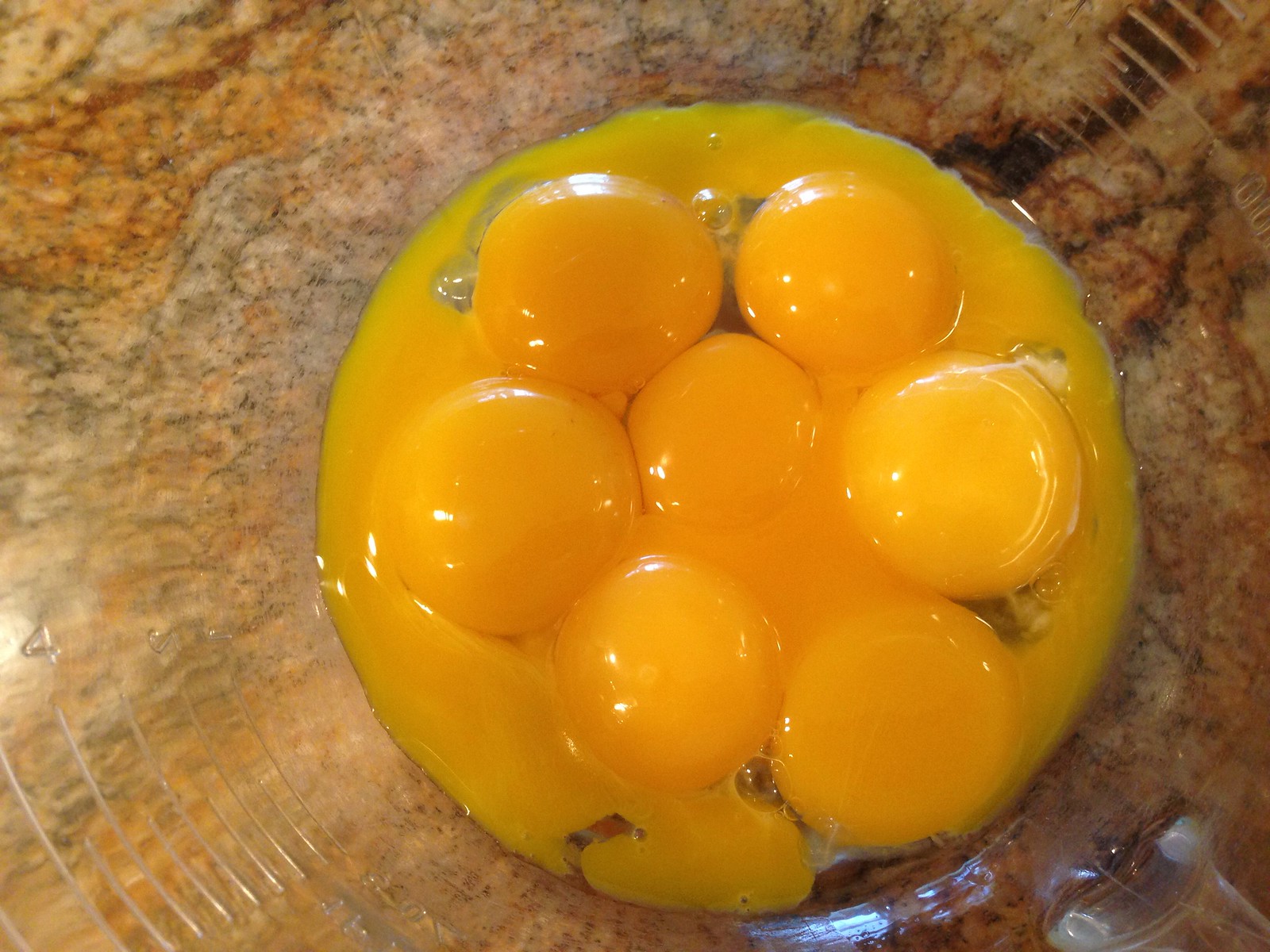The image is a close-up color photograph in a landscape orientation, looking straight down into a clear glass mixing bowl with ridges running concentrically around its circumference. The bowl is set on a multi-colored marble worktop, featuring a blend of red, pink, dark maroon, and other speckles. Inside the bowl, there are seven egg yolks, six arranged in a circle around a central one, with some yolks broken and their liquid mingling with the egg whites at the bottom of the dish. Highlights from lighting, possibly natural light or camera flash, reflect off the convex surfaces of the egg yolks. Additionally, the bowl includes a measuring scale with numbers visible on the left side (1, 2, 4) and a section of the scale visible at the top right.